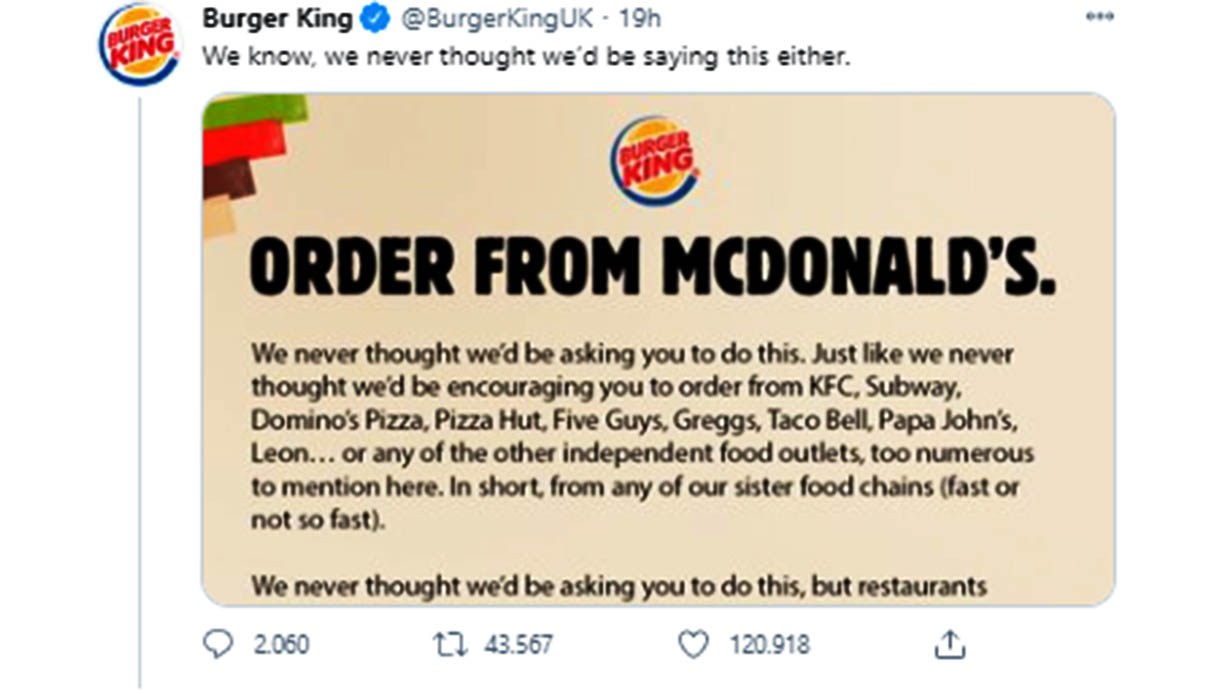The Twitter post is a notable announcement by Burger King UK, urging customers to order from rival food establishments, including McDonald's, KFC, Subway, Domino's, Pizza Hut, Five Guys, Gregg's, Taco Bell, Papa John's, Neon, and other independent food outlets. The post features the traditional Burger King logo in the upper left-hand corner, characterized by yellow top and bottom "buns," red "Burger King" text in between, and a blue outer trim. Accompanied by a blue verified checkmark, it reads "Burger King UK" followed by "19 hours." The tweet expresses an unprecedented solidarity with other food chains, acknowledging the challenging circumstances faced by restaurants. The image's text abruptly ends, leaving the latter part of the message incomplete. Engagement metrics below the post indicate substantial interaction, with 2,060 comments, 43,567 shares, and 120,918 likes.